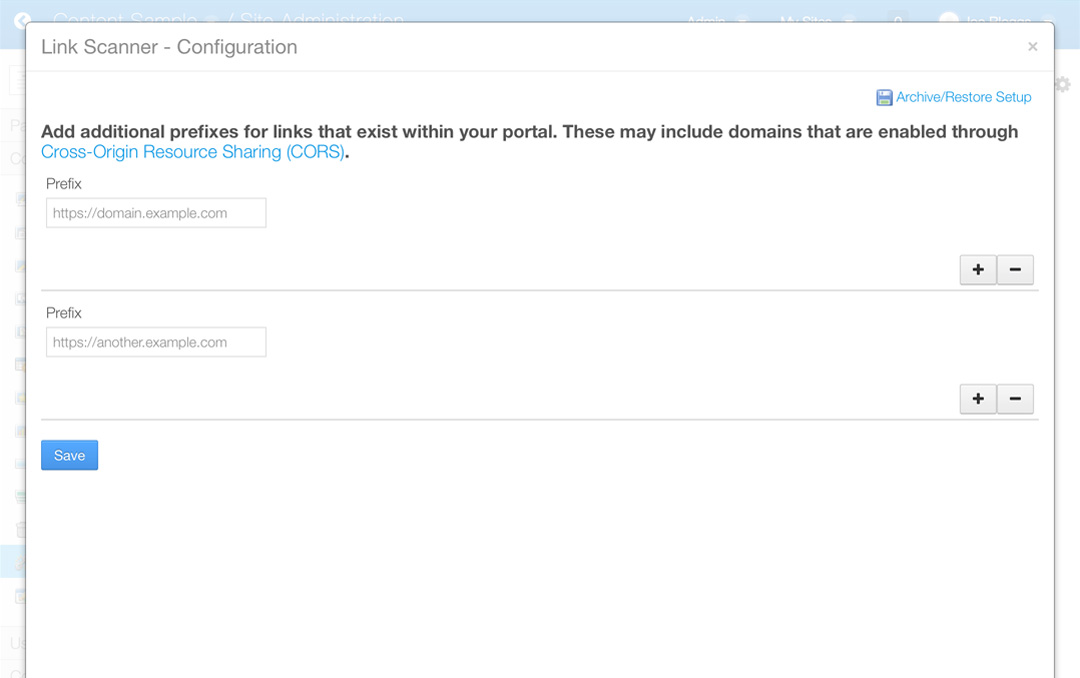Here is a detailed and cleaned-up caption for the image:

---

This is a screenshot displaying a web page in the background with a light blue bar. In the foreground, there is an inset page titled "Link Scanner - Configuration" at the top left. On the right side, there's an icon of a computer disk, followed by the clickable text "Archive/Restore Setup" in blue ink.

Below that, the page provides instructions in black ink: "Add additional prefixes for links that exist within your portal. These may include domains that are enabled through Cross-Origin Resource Sharing (CORS)." The term "Cross-Origin Resource Sharing (CORS)" is highlighted in blue, indicating it is a clickable link.

Further down, there is a labeled section "Prefix" with a text box containing "https://domain.example.com." To the far right of this text box, there are two light gray buttons: one with a plus (+) sign and another with a minus (-) sign.

Following this, there is another text box under the same "Prefix" label containing "https://another.example.com." Similarly, it has two light gray buttons to the right: a plus (+) and a minus (-).

At the bottom left of the inset page, there is a clickable blue button labeled "Save."

---